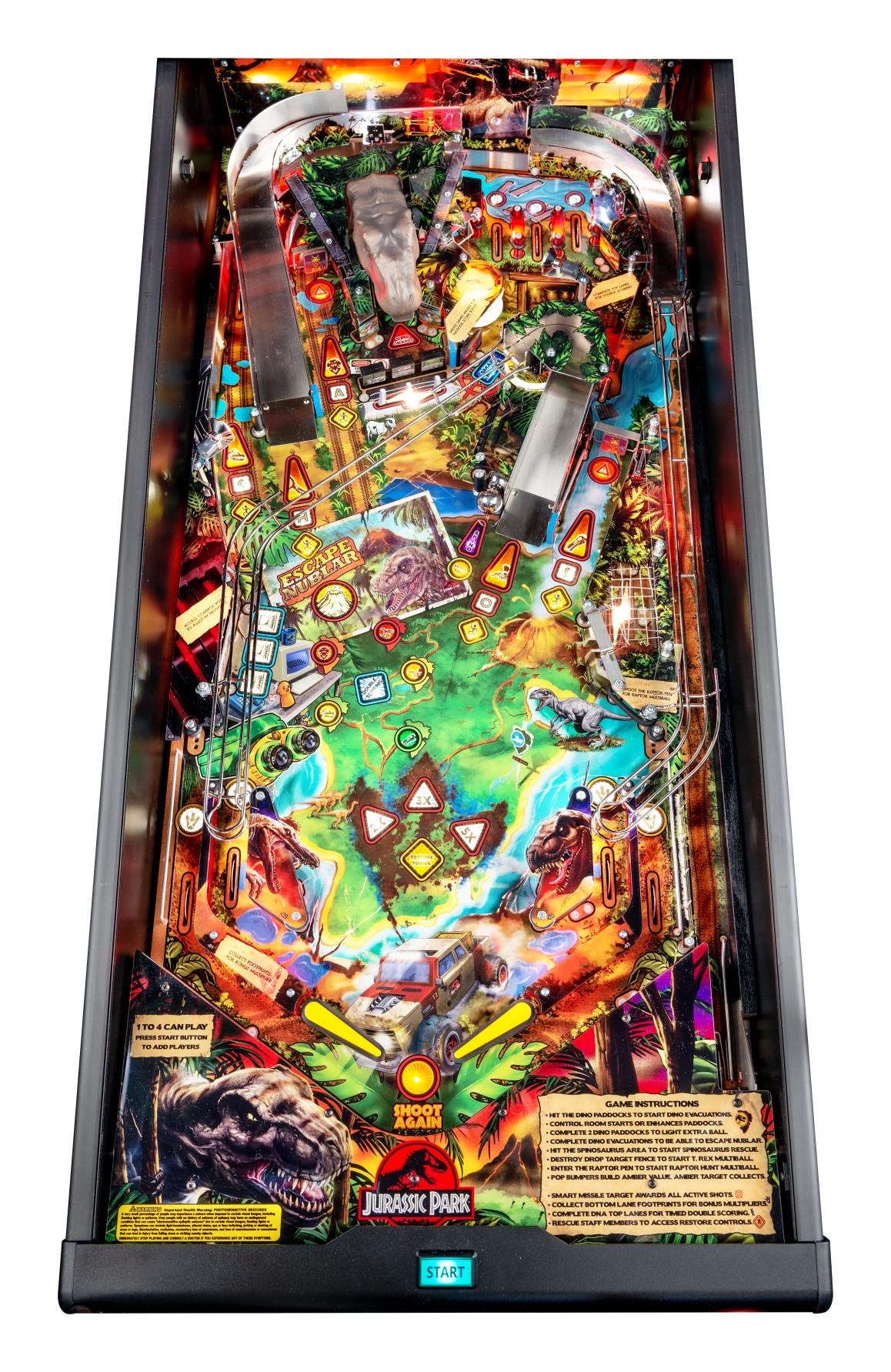This is a vibrant color photograph showcasing the playing surface of a Jurassic Park-themed pinball machine. The bottom section of the glass features a prominent label with the iconic Jurassic Park logo: a black silhouette of a dinosaur set against a red background, accompanied by white text that reads "Jurassic Park." Directly below, on the black frame of the machine, an illuminated blue square start button with black text stands out.

The design on the machine's glass includes instructions, though they are too small to be read in this image. The play area is vividly detailed, reflecting the Jurassic Park theme throughout. Bright yellow flippers are positioned at the bottom, ready to launch the ball, while a chute is visible on the right side to guide the ball's return. Various obstacles and pathways, characteristic of a pinball machine, add to the complexity and excitement. On the upper left side, a colorful chute where the ball emerges is noticeable.

Centrally located on the playing field is a green map of Jurassic Park, further enhancing the thematic immersion. This detailed design and vibrant color scheme make the Jurassic Park pinball machine a visually captivating and engaging experience.